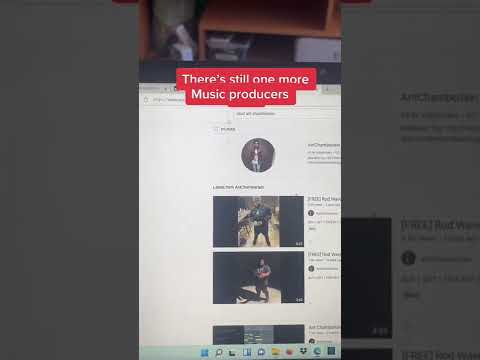The image presents a complex composition featuring two overlays of computer screens. The background appears to be a darkened photograph of a YouTube interface, identifiable by its white background and sequential video thumbnails. This background is slightly obscured, suggesting it was captured in a low-light setting or at an angle that reduces clarity, possibly indicating a handheld photo of a screen.

In the foreground, another image of a computer screen is superimposed, noticeably askew, indicating it’s a photograph rather than a direct screenshot. The edges of this foreground image reveal part of the monitor and the room behind it, making the setting of a physical space evident.

Adding to the scene’s complexity, a red text bubble with white text is prominently displayed over this foreground image. The text reads, “There’s still one more music producer,” suggesting a call-to-action or announcement. This design element, combined with the vertical video format, hints that the entire composition might be sourced from a TikTok video. The layering of images, text bubble, and the potential use of TikTok’s recognizable format contribute to the multimedia storytelling characteristic of the platform.